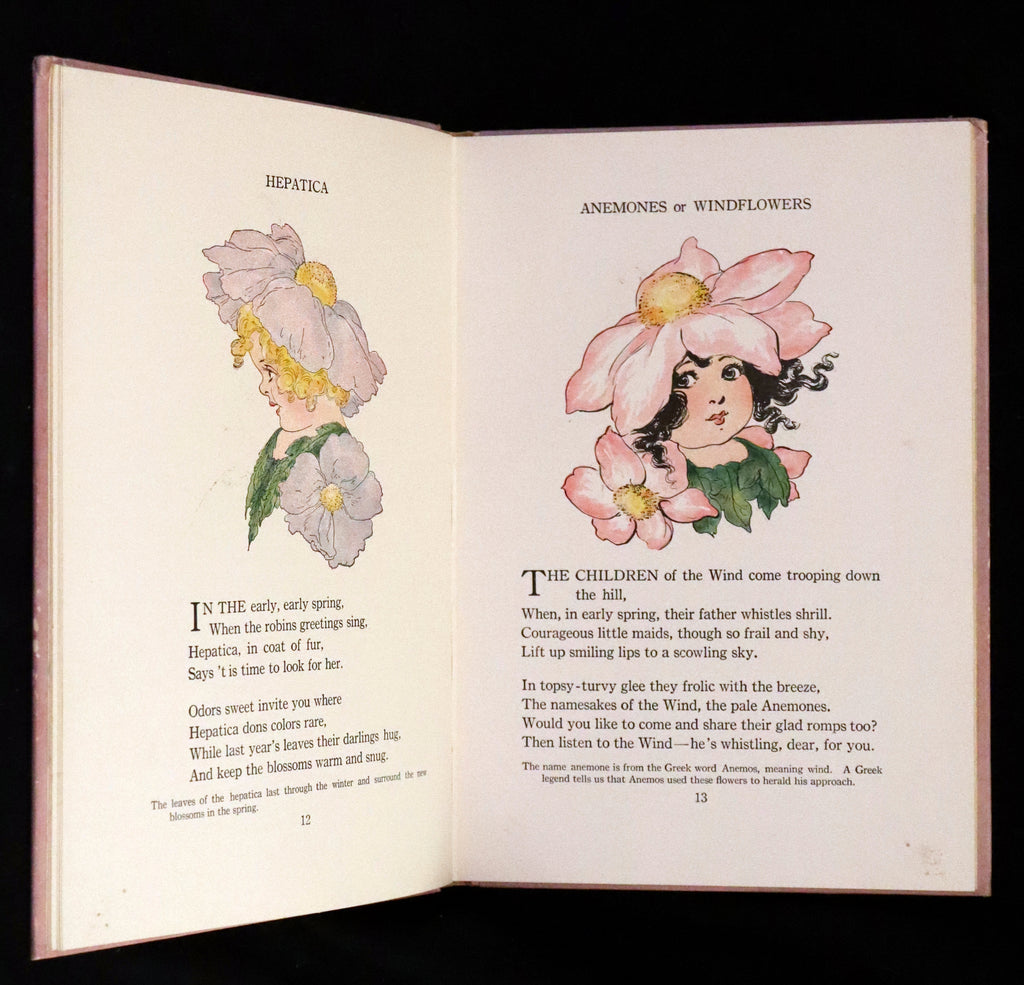The image showcases an open book set against a completely black background. The book's white pages feature illustrations and text in black ink. On the left page, the top text reads "Hepatica," and it displays the side profile of a little girl with golden, curly hair adorned with a floral hat resembling a flower with multiple petals. She also has a flower by her shoulder and is dressed in an outfit resembling green leaves. Beneath her image is a poem describing her, suggesting she symbolizes the Hepatica flower. On the right page, the text at the top reads "Anemone" or "Windflowers." This page features a little girl with curly black hair, facing forward with a chubby face. She wears a flower hat similar to the one on the left page, has a flower on each shoulder, although one is partially obscured. Her attire also appears to be fashioned from green leaves. Below her image is another poem, which elucidates the characteristics of the Anemone flower. Both poems explain the origins and meanings behind their respective flower illustrations.